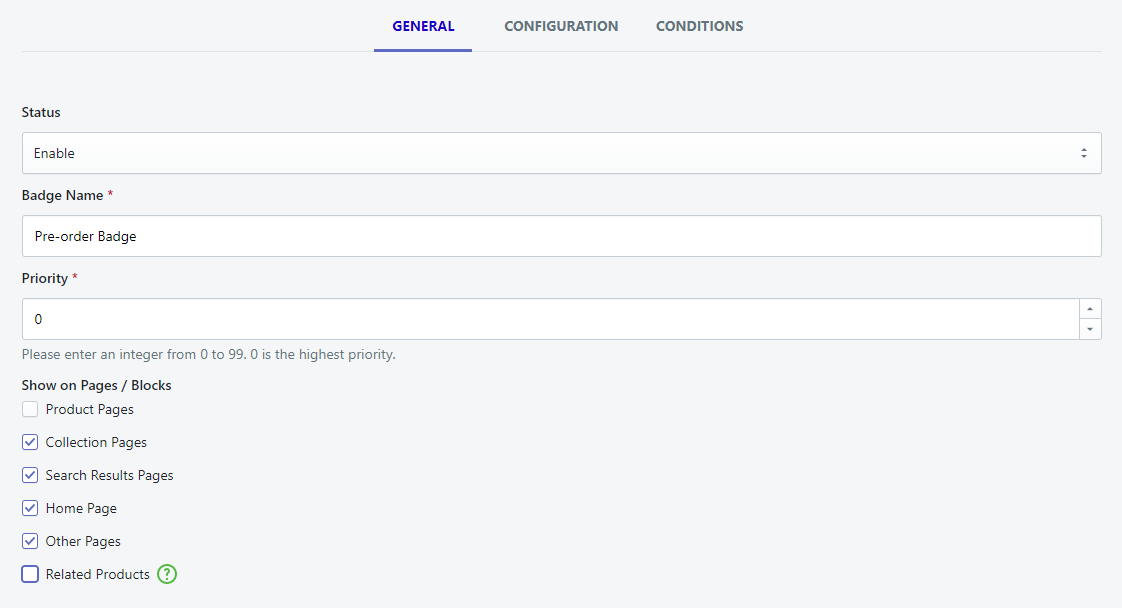In this detailed image, we observe a user interface with three distinct categories displayed prominently at the top center. The first category, labeled "General," is highlighted in purple, accompanied by a horizontal purple line beneath it, indicating it is the currently selected section. Adjacent to "General" on the right are the words "Configuration" and "Conditions," both rendered in light gray text.

Beneath these categories, multiple text fields are visible. Starting from the left, the first field is titled "Status," and directly below it is a boxed area containing the word "Enable." The right end of this box features up and down arrows.

Following the "Status" field is the "Badge Name" field, marked with a red asterisk indicating a required field. This box is labeled "Pre-Order Badge." Underneath this, the "Priority" field, also accompanied by a red asterisk, displays a default value of zero and includes up and down arrows on its right end.

At the bottom left corner of the image, there are several small checkboxes in varying states (checked or unchecked), indicating various options or settings related to the fields above.